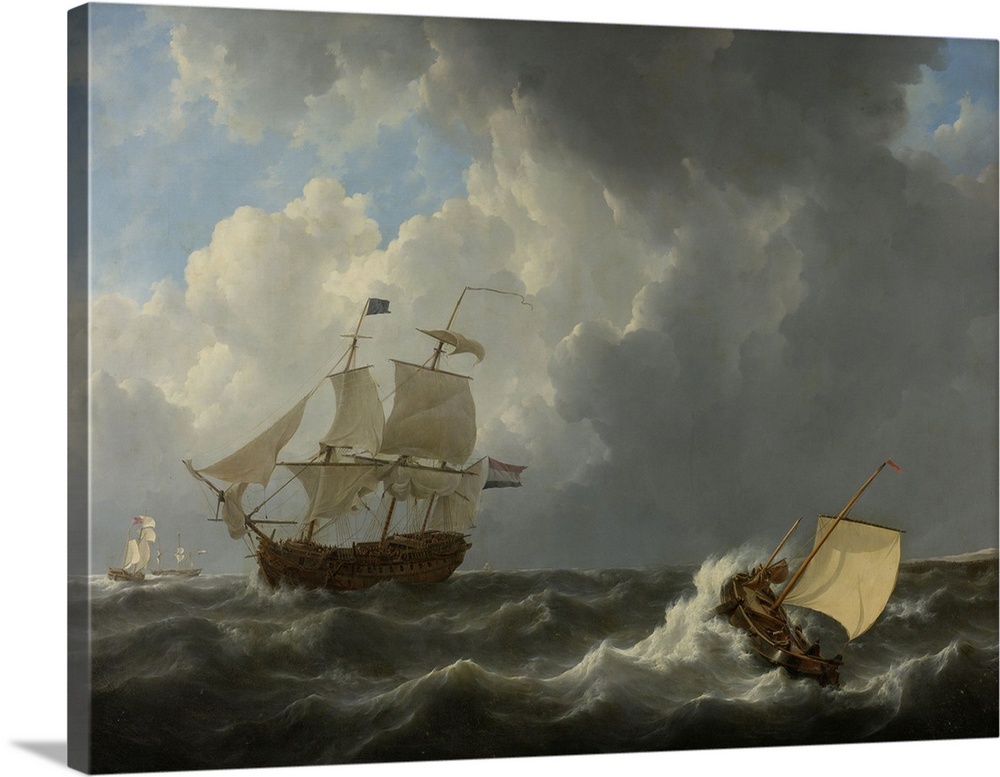This painting captures a dramatic scene of ships battling through rough seas. Dominating the scene, a large wooden ship with white sails, reminiscent of vessels from the 17th or 18th centuries, is positioned slightly to the left of center. The ship, facing leftward, features a hard-to-discern dark flag at its top, hinting at a possible pirate affiliation, while a more clearly visible red, white, and blue flag flies towards the rear. The turbulent waters are dark and choppy, a dark green hue reflecting the stormy conditions with waves cresting high. Surrounding the main vessel, two smaller ships can be seen further left in the background, tossed about by the rough sea. On the bottom right, a much smaller boat, with a single sail and crusted by a wave but seemingly intact, adds to the sense of chaos. The sky further enhances the ominous atmosphere with dark gray clouds, almost black, crowding most of the scene. However, patches of light blue sky peek through at the top left and right corners, offering a stark contrast to the stormy turmoil below. Some white clouds are also visible, adding layers to the sky’s texture and emphasizing the severity of the weather these ships are enduring.